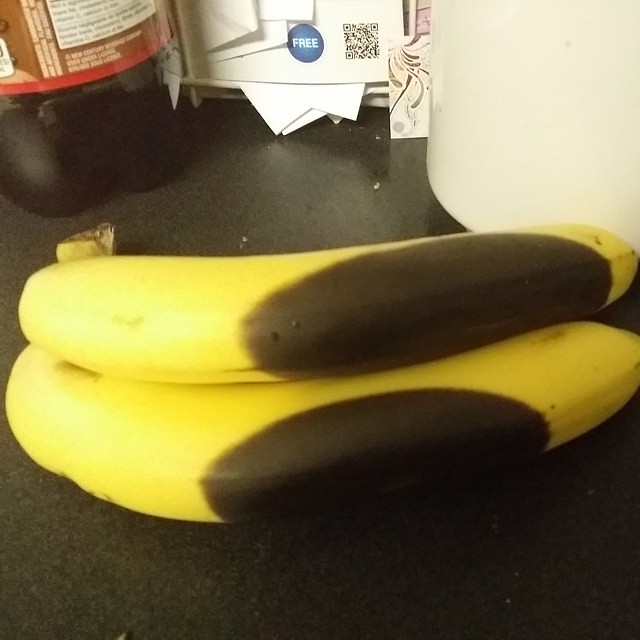This color photograph showcases a pair of yellow bananas lying horizontally on a black kitchen countertop. Each banana features a large, oval-shaped black spot on its peel, starting from about the midpoint and extending downward. The regularity and size of these black areas suggest they might be artificially created, possibly AI-generated. The curved sides of the bananas face the viewer, with one banana resting atop the other.

In the background, on the left, there is a bottle partially filled with a dark liquid, possibly root beer, given its reddish-brown label with white writing. Adjacent to the bottle, various pieces of paper are overlapped. One of these papers bears a round blue logo with the word "free" in white and a QR code beside it. Another piece of the paper appears pink with black squiggly lines. In the upper right corner, the curvature of a large white round object, likely a canister, is partially visible. The lower corners of the photograph are engulfed in shadow, drawing further attention to the prominently featured bananas with their unusual discoloration.